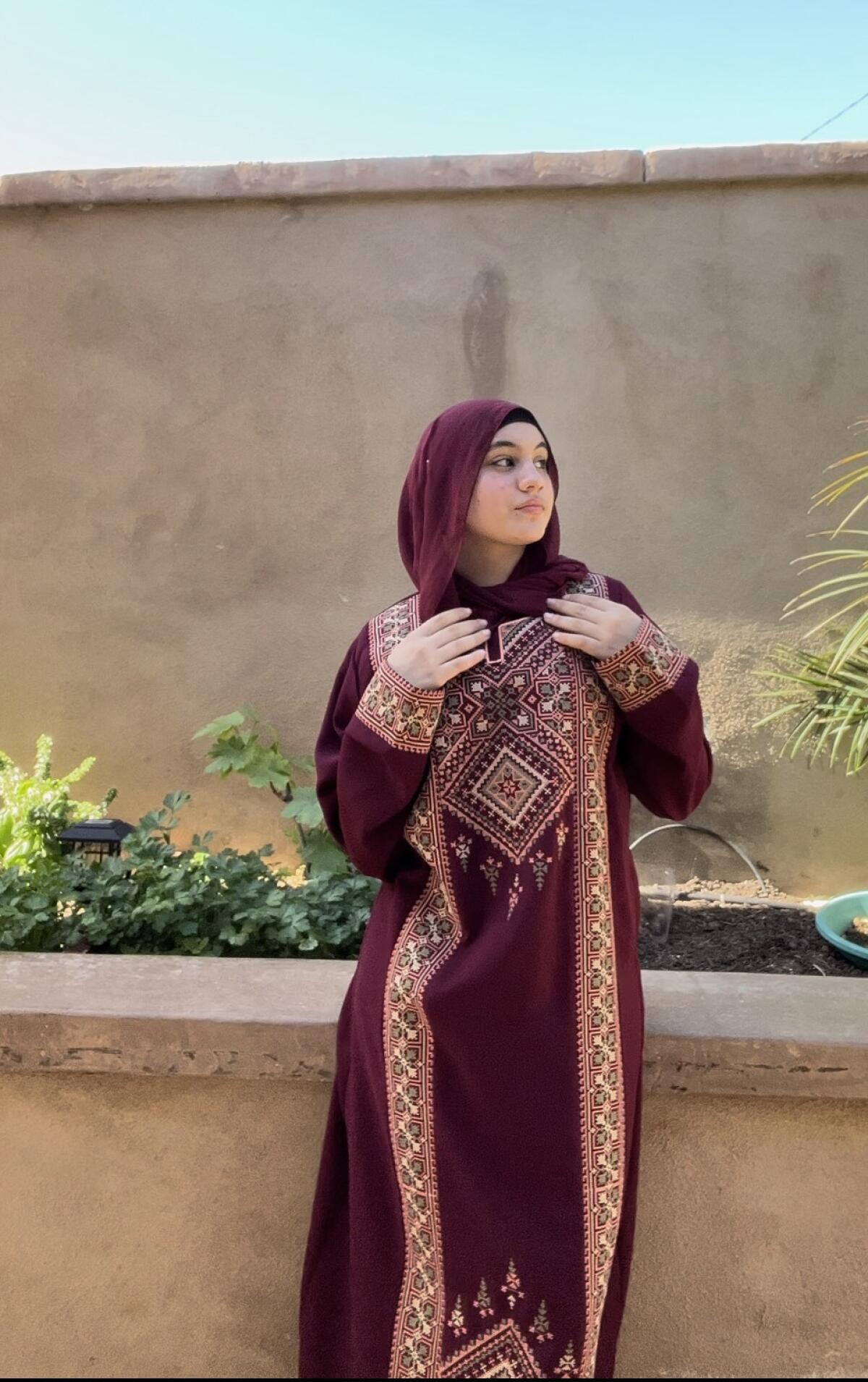The image features a young woman standing against a waist-high, tannish stone wall, with soil and plants visible behind her. She dons a long, maroon-colored dress, intricately adorned with a detailed, ornate pattern featuring hints of tan, pink, and green along the front and sleeves. Her maroon head covering conceals her hair, and she looks off into the distance to her left with a neutral expression. Her hands rest close to her shoulders. Behind her, a much taller wall, around 12 feet high, rises towards a clear, bright sky. The photo, in portrait orientation, captures her from head to about her calves, emphasizing the soft sunlight and serene backdrop.